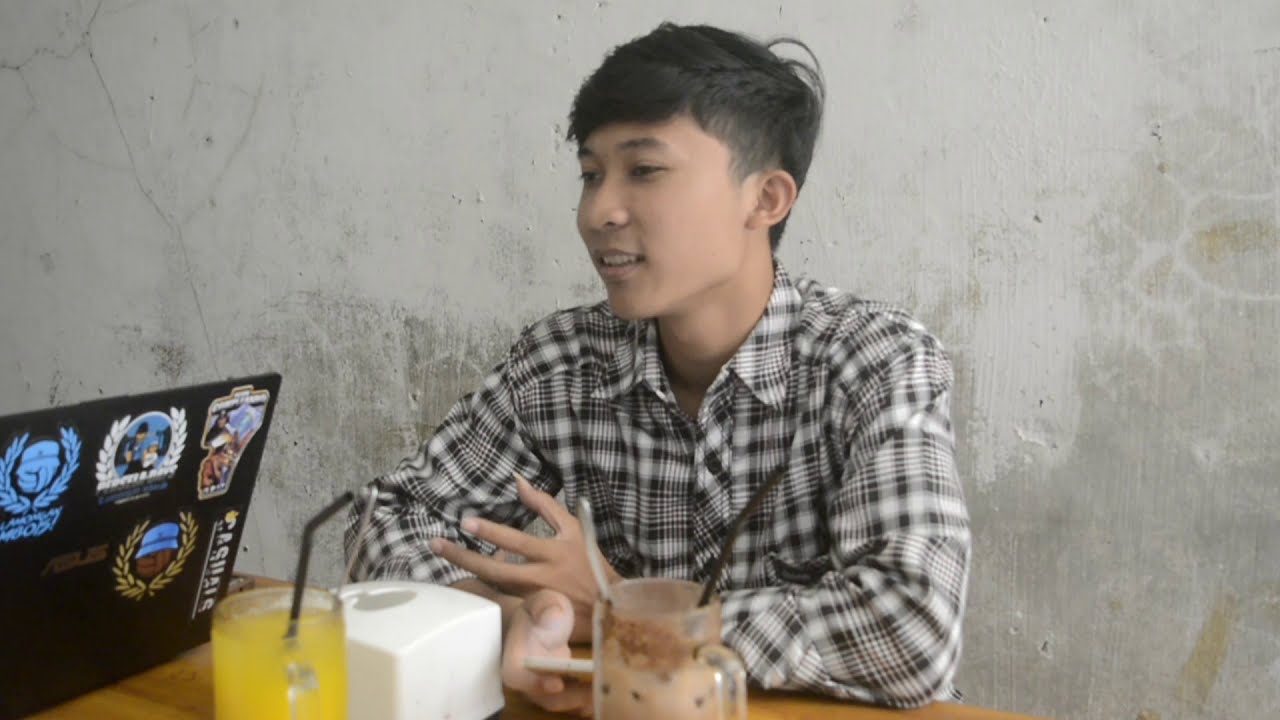The photograph captures a young man, possibly a teenager, with dark hair and a noticeable cowlick, sitting at a wooden table. He is wearing a long-sleeve black and white plaid shirt with the top button undone. Behind him stands a concrete wall showing some discoloration. He is seated with his elbows propped on the table and looking off to his right, seemingly in the midst of explaining something. In front of him, there's a white plastic box and two glass mugs; one seems to have held a milkshake with a spoon and a straw sticking out, while the other contains an orange-colored drink with a black straw. To his right, there is an open black Asus laptop adorned with several stickers. The scene clearly takes place indoors, in a shaded setting, likely in a casual or informal environment.